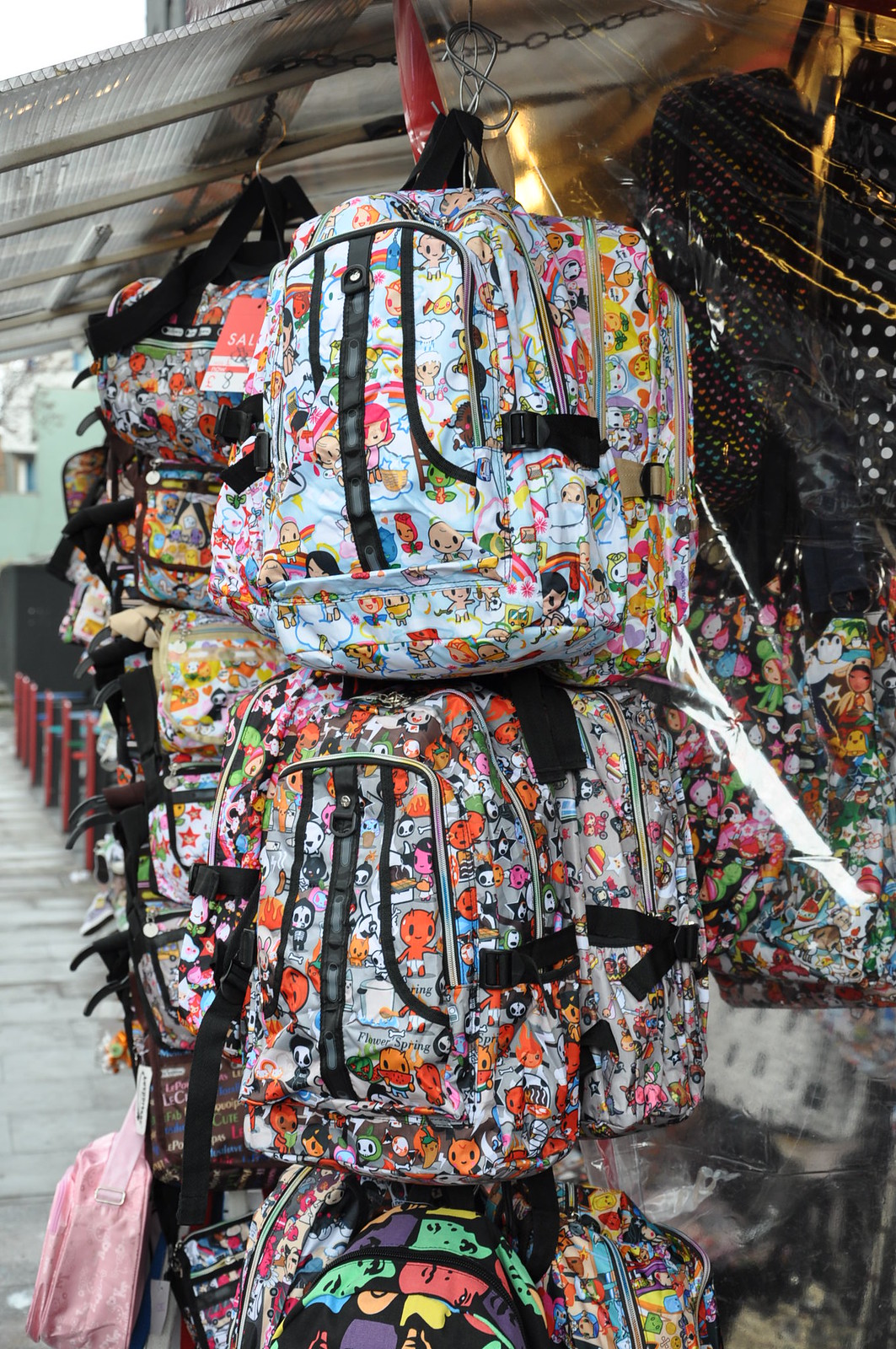This vibrant photograph captures an array of brightly colored children's backpacks hanging from hooks under a fabric canopy, typically seen in open-air marketplaces in East Asia. The vendor stall is vividly decorated with these vinyl backpacks, each adorned with intricate cartoon characters and diverse playful designs. Among them, one backpack stands out with a light blue background featuring various cartoon figures, while another, slightly spiritual in theme, has a light grey base with "Flower Spring" text inscribed on it. These backpacks evoke a distinct anime feel, with designs including cute, colorful angels, flowers, and equally enchanting devils alongside chili peppers and skeletons. The backdrop subtly hints at a broader marketplace scene, with a blurry seating area to the left, suggesting a nearby food hall or cafeteria. The top right-hand corner features polka dots, adding to the overall whimsical aesthetic.